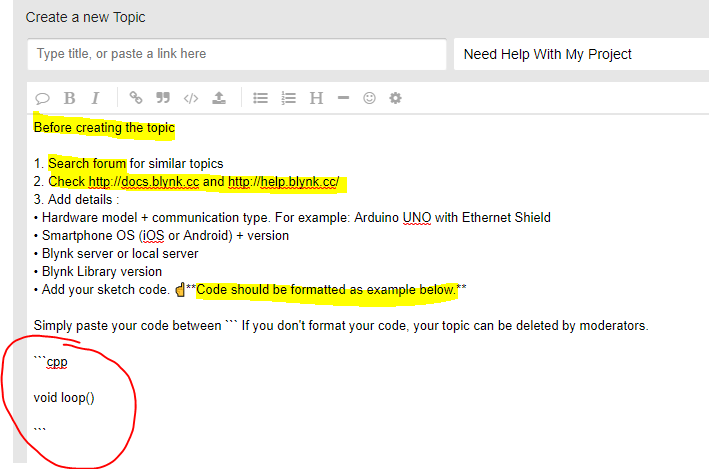This is a screenshot of a web page dedicated to creating a new topic. At the top, there is a gray header with the prompt "Create a new topic" prominently displayed. Down the left side, a gray border frames the page. Below the header, a white input box labeled "Type title or paste a link here" is visible, followed by the text "Need help with my project" within another white input field.

The main body of the page features zones of varying shades of gray and white, creating a clear visual hierarchy. At the very top, iconography is utilized alongside text instructions. Highlighted in yellow, the first instruction reads, "Before creating the topic, search the forum for similar topics." The term "search form" is also emphasized in yellow. 

Following this, a numbered list of steps guides the user through the process: 
1. Search the forum for similar topics (highlighted in yellow).
2. Check referenced websites provided.
3. Add details about the hardware model and communication type, with examples such as "smartphone OS: iOS or Android plus version, Blink server or local server, Blink library version."

The section outlines how to add sketch code, providing a formatted example and emphasizing the importance of proper code formatting to avoid topic deletion by moderators. This instruction is illustrated by a red circle highlighting the example code snippet: "dot dot dot CPP avoid loop."